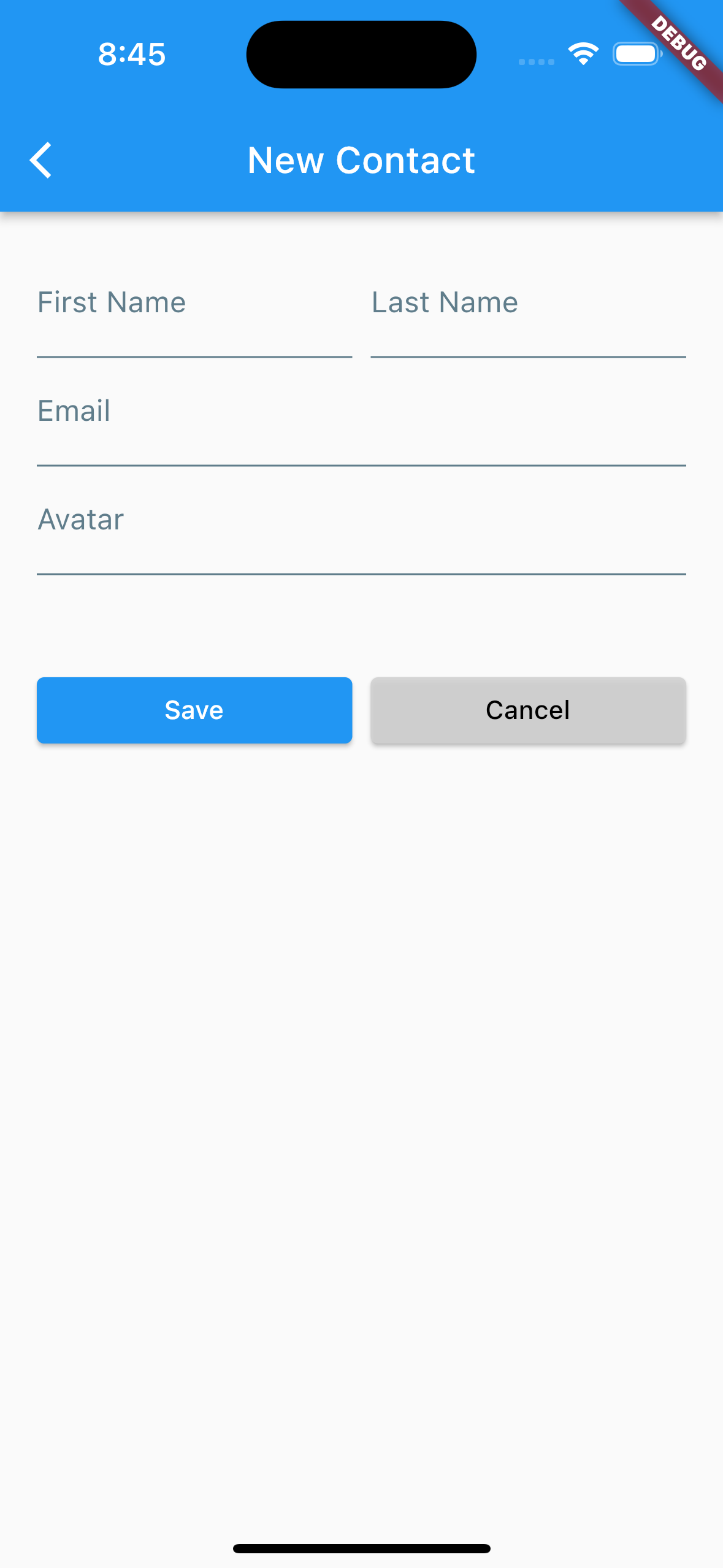This is a screenshot of a smartphone displaying a user interface, likely from a mobile application or website in a beta or debug phase. The device's status bar indicates the time is 8:45 (AM or PM is indeterminate) and shows a fully charged battery icon. A distinct red banner labeled "DEBUG" diagonally spans the top right corner, suggesting that the interface is in a testing mode.

The main content of the screenshot is a form for adding a new contact, indicated by the "New Contact" title centered at the top of the screen. There is a back arrow in the top left corner for navigation. The form fields are organized as follows: at the top left are the "First Name" and "Last Name" input fields side by side. Below these is an "Email" field, followed by an "Avatar" field, which might be intended for a username or alias rather than a profile picture. At the bottom of the screen, there are two actionable buttons: a "Save" button on the left and a "Cancel" button on the right.